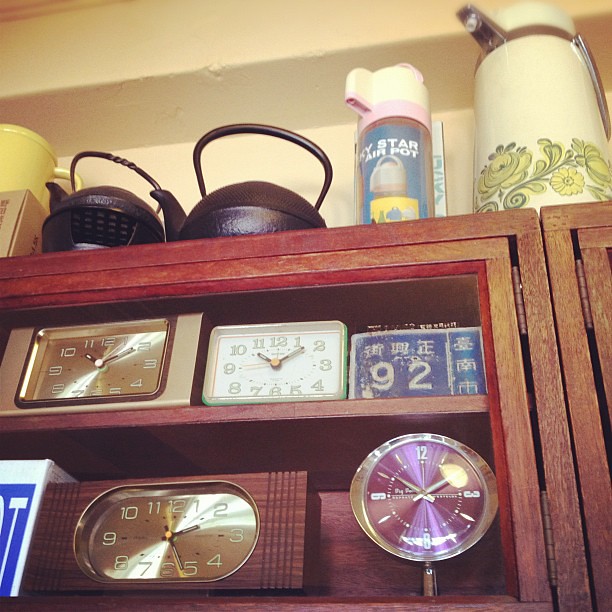A detailed image showcasing a cozy, rustic section of a small general or hardware store, focusing on a brown wooden shelf unit with hinged doors. The bottom two shelves are populated with a variety of clocks, each differing in shape, size, and color. Some clocks gleam with metallic finishes while others are designed with colorful plastic casings. The top shelf features a pair of black kettles, with one noticeably larger than the other. Alongside the kettles, two distinct vacuum flasks are displayed: one is cream-colored adorned with a delicate pattern of green foliage and yellow flowers, while the other is a vibrant mix of blue, white, pink, and yellow hues. The arrangement exudes a nostalgic charm, blending practical household items with vivid, eye-catching designs.